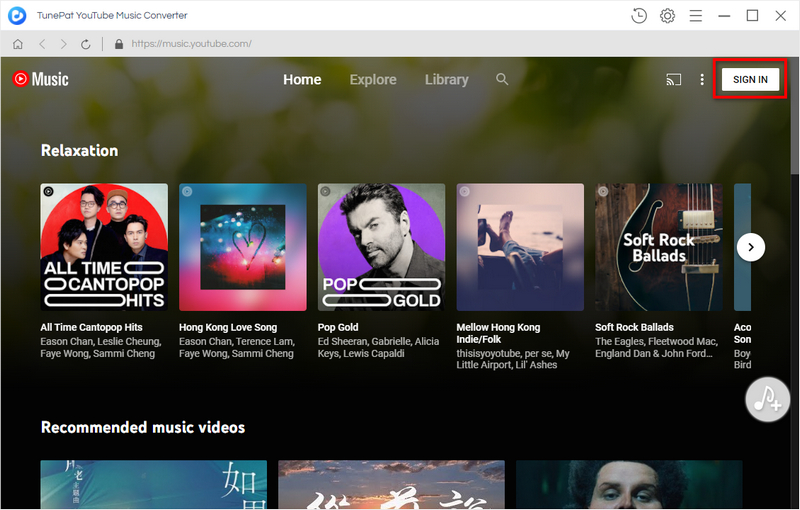This image is a detailed screenshot of a computer screen displaying the ToonPat YouTube Music Converter interface. In the top left-hand corner, a logo is followed by the text "ToonPat YouTube Music Converter." On the right side of the top bar, there are icons for refresh, tools, minimize, maximize, or close the window.

Below this top bar, there is another toolbar containing a home button, forward and back navigation buttons, a refresh button, and a search bar. The left side of the toolbar displays a menu with options like Music, Home, Explore, Library, and Search, accompanied by icons. The Home option is highlighted. On the right side, there is a white "Sign In" button outlined in a red square for emphasis.

Beneath this toolbar, multiple album covers are displayed. From left to right, the albums are titled "All Time Canto Pop Hits," "Hong Kong Love Song," "Pop Gold," "Mellow Hong Kong Indie Folk," and "Soft Rock Ballads." A right arrow allows users to scroll through additional albums.

Further down the screen, a section labeled "Recommended Music Videos" shows the top third of three music video thumbnails. The captions or titles of these videos are not fully visible, though some feature text in Chinese or Korean.